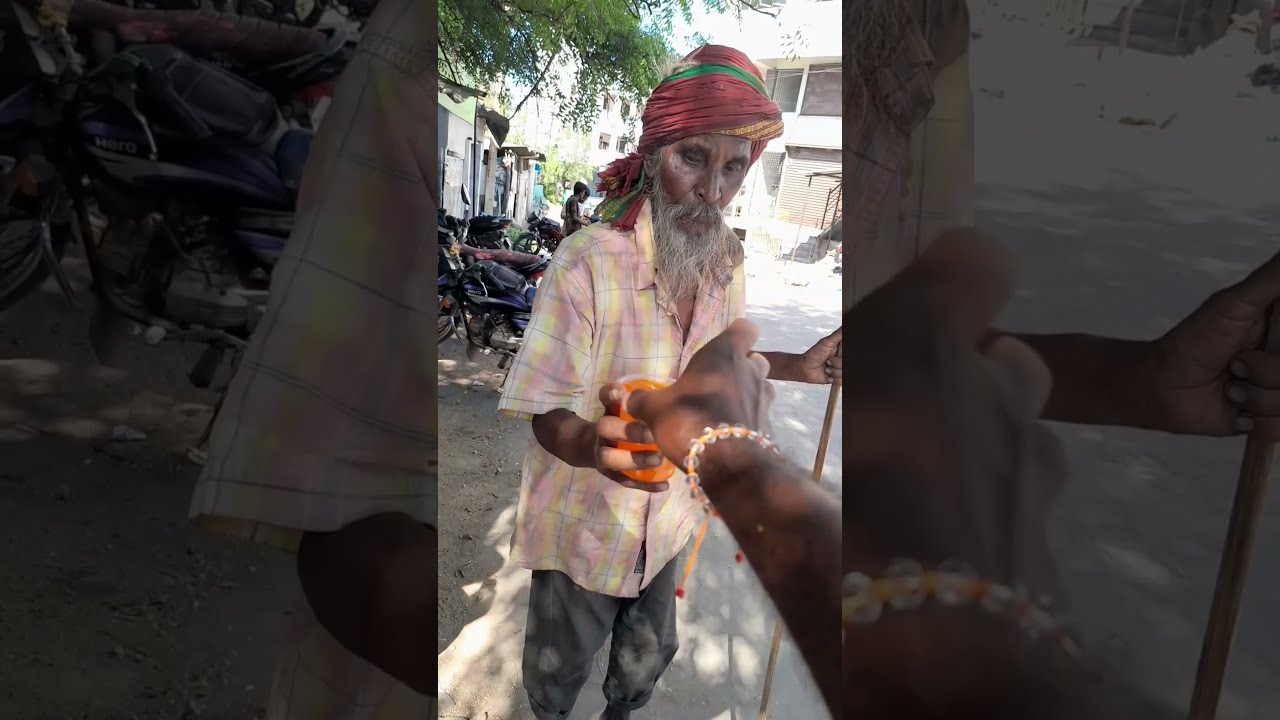In the center of the image, a vertical cell phone style photo captures an elderly Indian man with dark brown skin and a long gray beard. He is adorned with a multicolored turban, primarily red with a green stripe, and wears a button-up short-sleeved shirt in pink and yellow hues that reaches his elbows. The man gazes downward towards his hand as he reaches out to accept a glass filled with an orange substance from another person with dark brown skin, who is wearing an orange and white bracelet. The man's other hand grips a wooden rod. The background showcases buildings, tables, and a tree, suggesting an outdoor, public setting in the middle of the day with a concrete surface. The left and right sections of the image are tinted and feature zoomed-in details: the left focuses on the man's elbow and shirt, while the right highlights the extended hand and bracelet. The image is detailed and vibrant, emphasizing the interaction and surrounding environment.